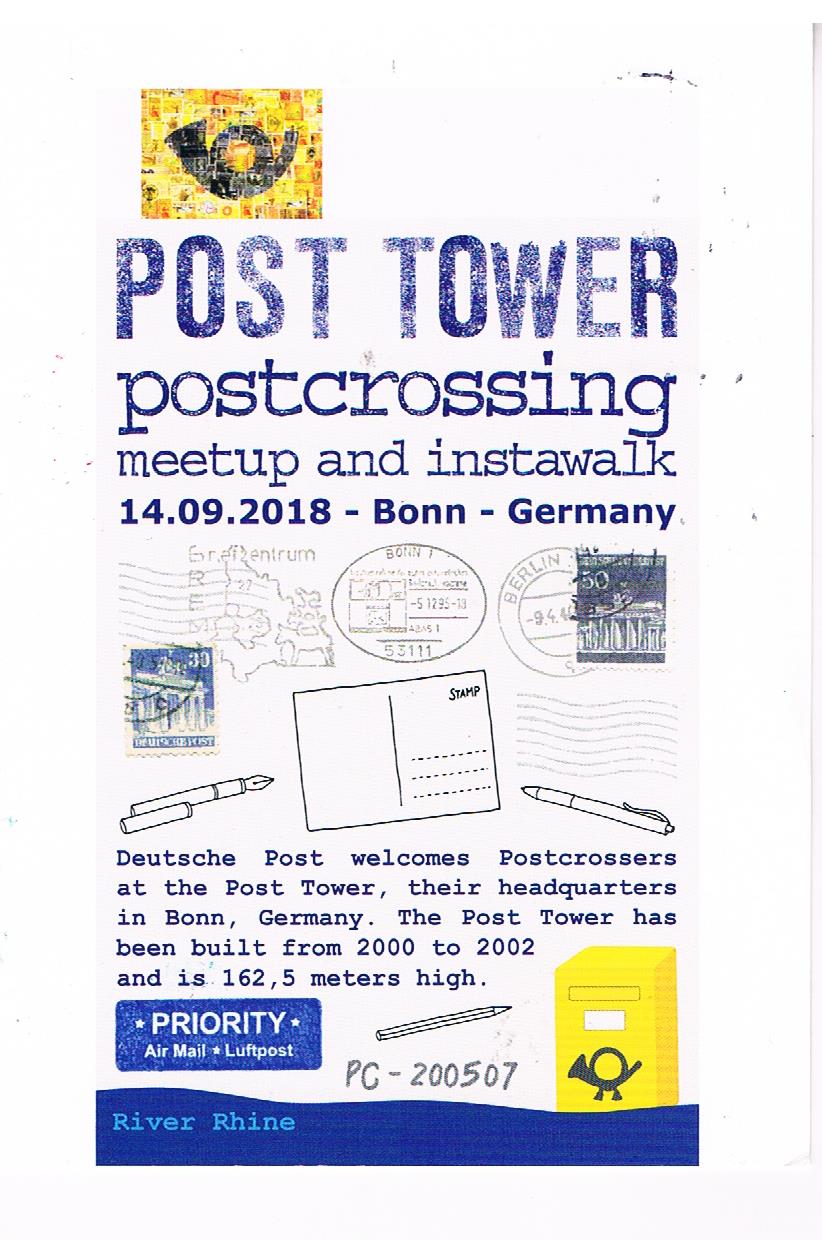This creatively designed flyer on a white background commemorates a Post Crossing meetup and instawalk at the Post Tower on September 14, 2018, in Bonn, Germany. The top left corner features a yellow rectangular icon with a collage of pictures forming a black trumpet-like shape. Below this, the headline "Post Tower" is prominently displayed in bold blue fonts, followed by "Post Crossing Meetup and Instawalk, 14.09.2018, Bonn, Germany." 

Further down, the text "Deutsche Post welcomes post crossers at the Post Tower, their headquarters in Bonn, Germany. The Post Tower was built from 2000 to 2002 and stands 162.5 meters high" appears in blue. Surrounding this text are various images, including maps of Germany, stamps featuring numbers and codes such as "53111" and "944 Berlin," a black-and-white pen and pencil, and a stock postcard labeled "Stamp" in the upper right. 

Additional elements include a yellow mailbox on the right with the same trumpet logo from the top left, and the text "Priority Air Mail, Luft Post" next to the pencil with the code "PC-200507" inscribed below it. A horizontal blue strip at the bottom bears the text "River Rhine." This flyer combines vivid illustrations and informative text, capturing the essence of this special event at the Post Tower.